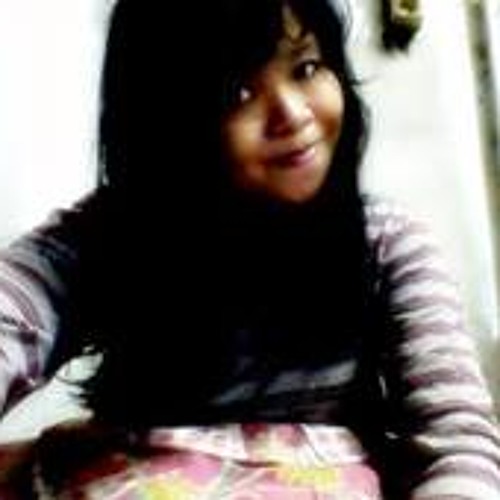In this low-resolution, blurry image, a Latina woman with long, dark hair and dark eyes is positioned at the center, slightly tilting her head to the side as she smirks or eyes the camera. Her facial features appear smooth due to the poor image quality and compression artifacts. She wears red lipstick and a long-sleeved, multicolored striped shirt predominated by lavender and dark purple hues. She sits in front of a door, with a lock visible just above her head. Her lap appears to hold a colorful object, possibly a floral or strawberry-patterned blanket, in shades of pink and yellow. The background details are unclear due to the image's low quality, making it hard to discern precise details about the setting.